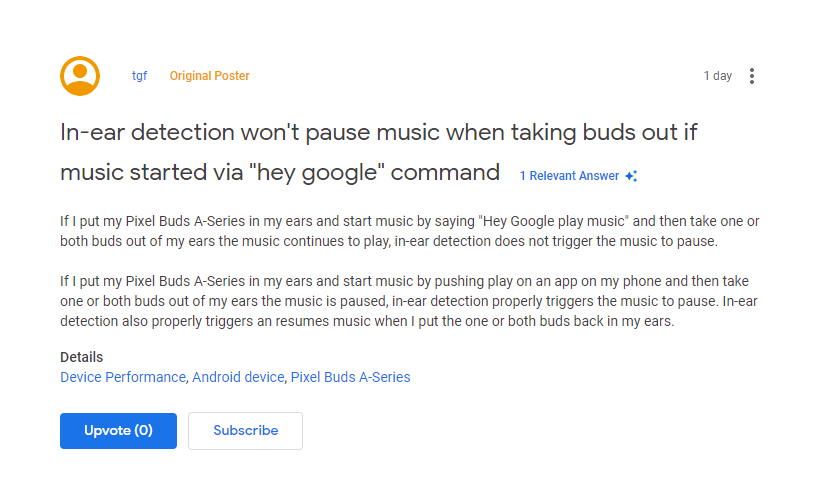This image is a detailed screenshot of a computer screen displaying a forum post. On the left-hand side, there is a circular icon featuring a person's silhouette, which represents the user. Next to this icon, the text "TGF" appears in blue, indicating it is a clickable link. Following that, the label "Original Poster" is highlighted in an orange-yellow color. On the far right, the timestamp "one day" is visible, accompanied by three vertical dots used to expand a menu.

Beneath these identifiers, the main content of the post begins with the statement: "In-ear detection won't pause music when taking buds out if music started via Hey Google command." This is followed by the heading "One relevant answer."

The content continues with two distinct paragraphs. The first paragraph states: "If I put my Pixel Buds A-Series in my ears and start music by saying 'Hey Google, play music' and then take one or both buds out of my ears, the music continues to play. In-ear detection does not trigger the music to pause."

The second paragraph clarifies: "If I put my Pixel Buds A-Series in my ears and start music by pushing play on an app on my phone and then take one or both of the buds out of my ears, the music is paused. In-ear detection properly triggers the music to pause. In-ear detection also properly triggers and resumes music when I put one or both buds back in my ears."

Following this explanation, there is a section labeled "Details" with a blue clickable link that reads, "device performance Android device Pixel Buds A-Series."

On the left-hand side of this section, there's an upvote button. To the right of this, next to the main content, is a subscribe button.